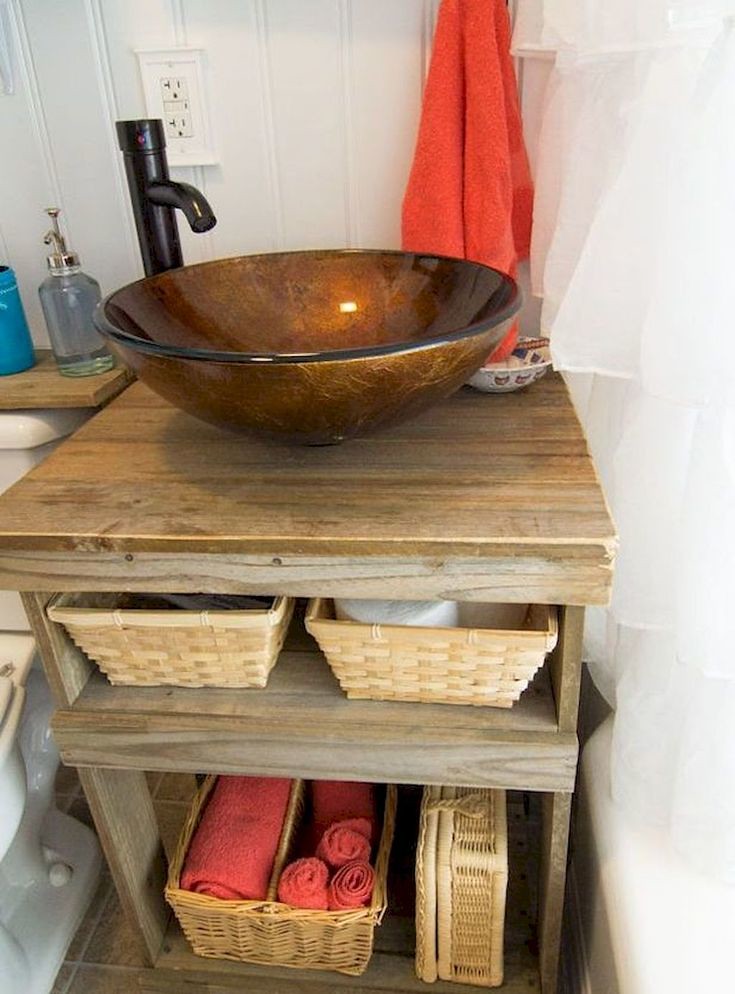The image depicts a rustic kitchen scene featuring a wooden cabinet. The cabinet comprises two shelves: the lower shelf is taller and houses two wicker baskets. The basket on the right is positioned sideways and has its lid closed, while the basket on the left is upright with rusty-colored towels neatly rolled up inside. The upper shelf also contains two open wicker baskets—one on the left with a partially visible gray or brown item, and one on the right with a partially visible white item.

Atop the cabinet sits a distinctive basin style sink, designed to resemble a bowl, with a pump tap extending over it. The background features a white wall with an electrical outlet. To the right, a towel hangs from the wall beside a window adorned with ruffled white curtains. On the left side of the image, a ceramic basin is visible, along with a shelf that holds what appears to be hand soap.